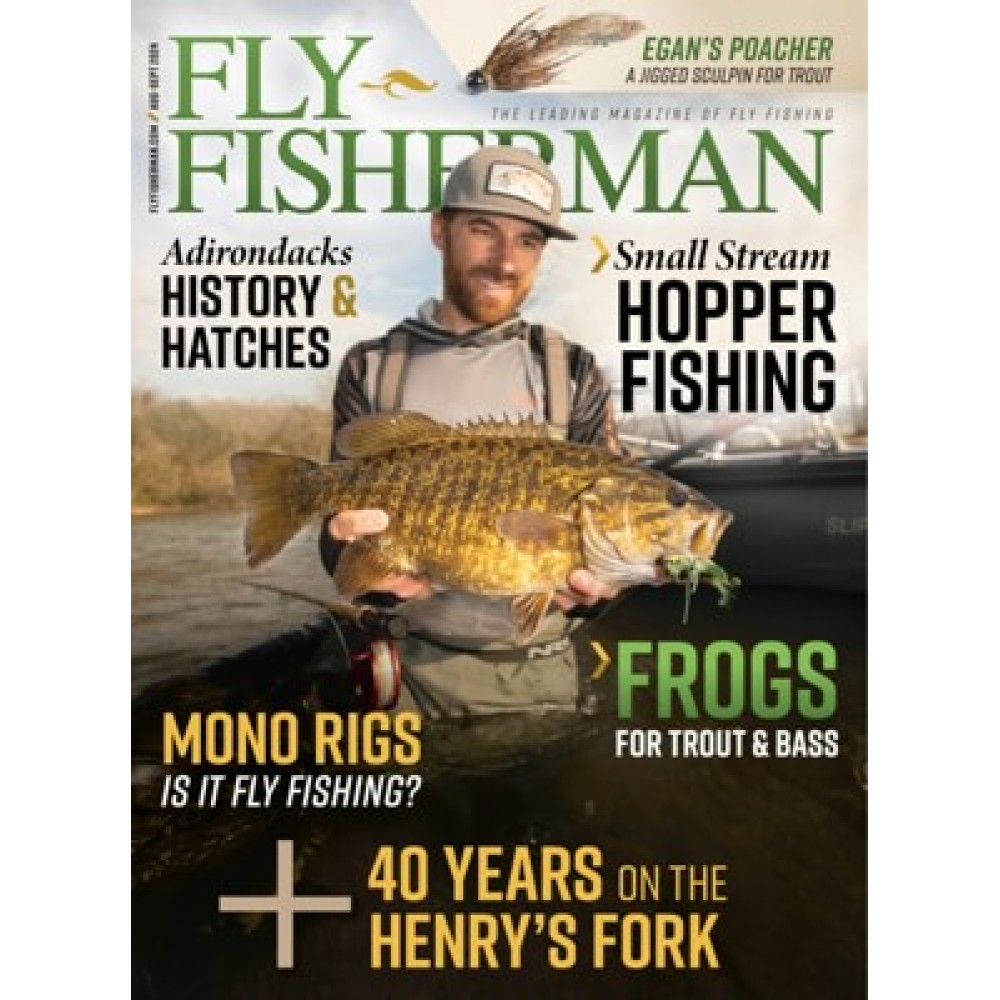The cover of Fly Fisherman magazine features a striking photograph of a man in shallow water, donned in a gray baseball cap with a camo pattern and an army-style brown jacket with a scarf around his neck. He proudly holds a large gold fish with black specks, approximately 15-16 inches long, which he lifts just above the water's surface. The magazine's title, "Fly Fisherman," is prominently displayed at the top in large yellow letters. Surrounding the man are various article titles, including "Gear Guide 2022 Award Winners Inside," "George Daniel Euro Jigging with Streamers," and "Silver Creek Better Than Ever." Additional highlighted features mention "South Platte Classics: RS2, Brassy, Miracle Nymph, Buckskin," and a peculiar note at the bottom reads "Guiding Martin Luther King" in yellow letters. In the upper right corner, the phrases "Hipster Doofus," "Kramer-approved," and "Carp-certified" add a quirky touch to the visually captivating and information-rich cover.